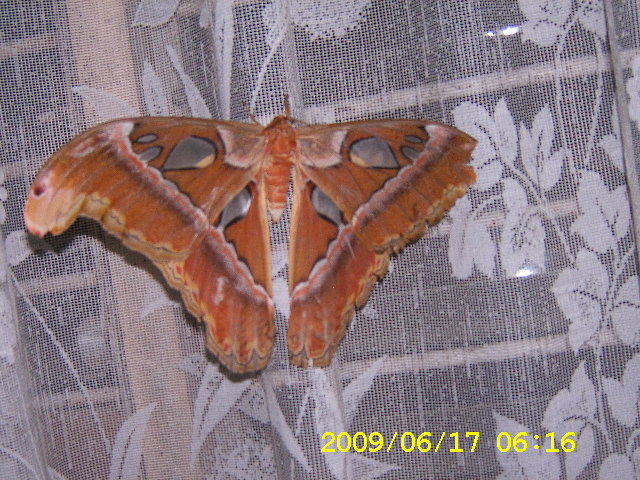This wide rectangular photograph captures a large moth, positioned just to the left of the center on a surface adorned with intricate white lacy fabric. The fabric features thick white leaves drawn on vines that extend upward on the right side and toward the left. The moth's orange, pointy body is oriented upward, and its wings are spread out symmetrically. These wings exhibit a complex pattern of orangey-brown hues with red, white, and black accents. Notably, there are gray spots, resembling holes, that give the impression of transparency and lead to darker borders that outline the wings. Additionally, subtle silvery teardrop patterns with dark borders enhance the delicate wing detail. A small white spot appears near the tip of the moth's tail. The bottom right corner of the image displays a timestamp in bright yellow, reading "2009-06-17 06:16."